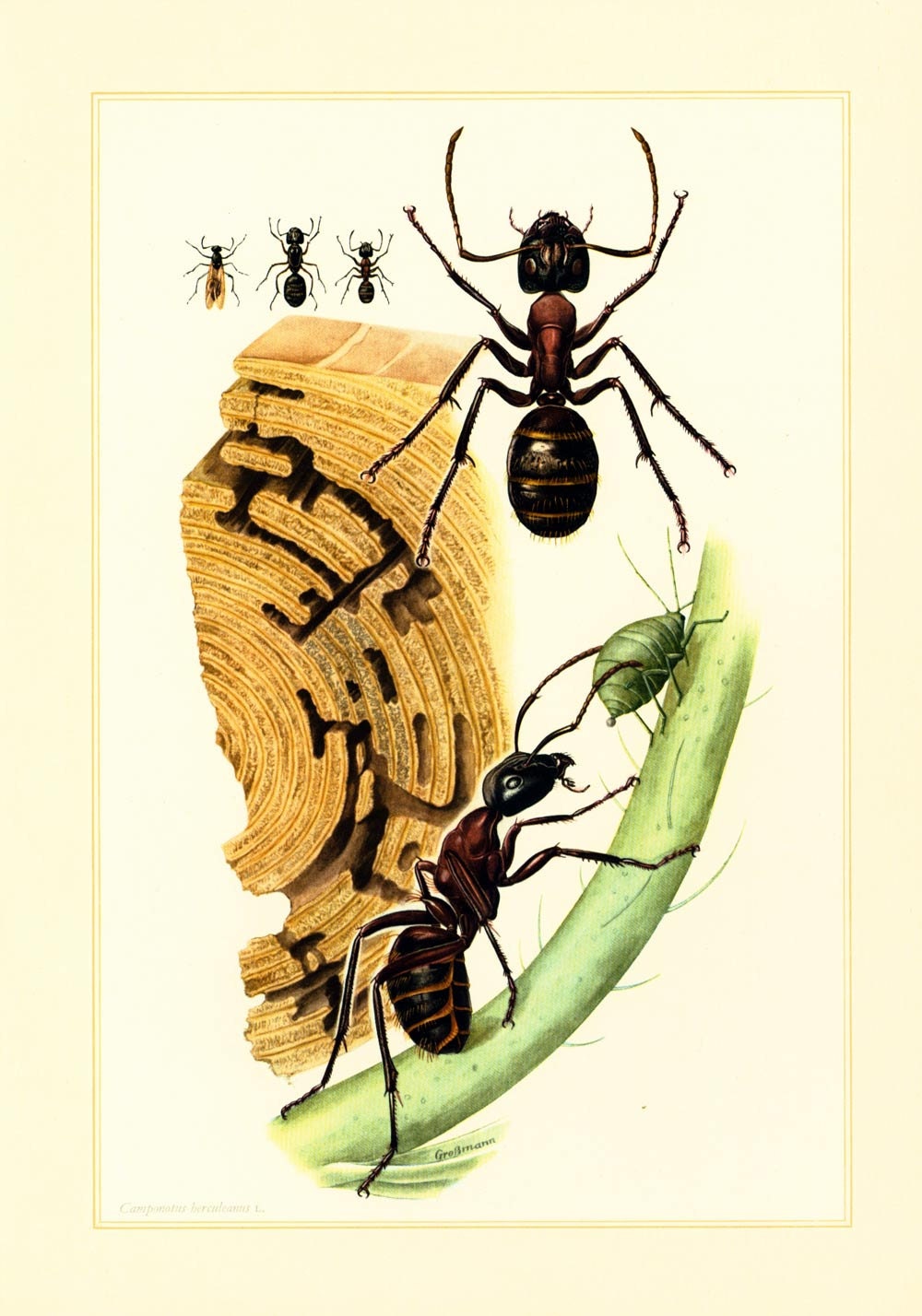The image seems to be a vintage-style diagram, framed by a yellow pastel border, depicting various ant-related elements. The background is a light lemon cream color, giving the illustration an older, classic appearance. In the top-left corner, there are three small ant illustrations, showcasing potential different types of ants. Adjacent to these, on the top right, is a significantly larger depiction of an ant, about ten times the size of the smaller ones, highlighting intricate details like its black and red body, eyes, antennae, and leg spikes. Below the smaller ant illustrations lies an image of intricately connected patterns, possibly illustrating ant tunnels within a tree stump, resembled to crop circles due to their elaborate design. To the right of this, near the bottom center, another detailed scene features an ant gripping a smaller bug, likely an aphid, on a flower stalk. This ant appears side-on, emphasizing its interaction with the aphid. Finally, the artist's signature is found at the bottom left, adding a personal touch to the detailed and educational illustration.